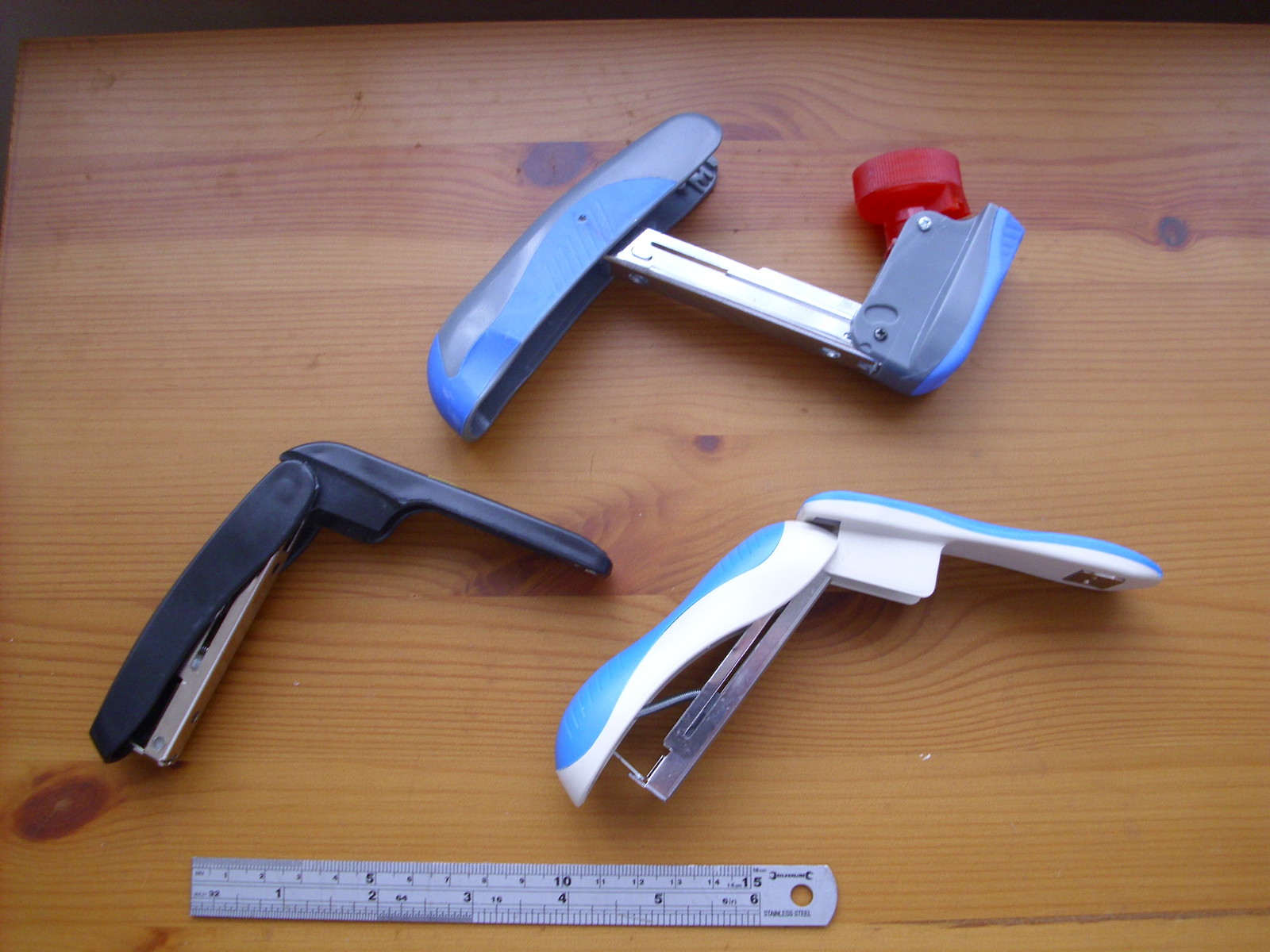The image displays three small, handheld staplers arranged almost in a triangular formation on a light brown wooden table with visible wood grain. Each stapler is open, revealing their empty interiors. At the top of the image, there is a light blue plastic stapler with an additional red component resembling a bottle cap. The bottom left has a simple black stapler, while the bottom right features a dual-colored stapler, primarily powder blue with white accents. Below the staplers, a metal ruler measuring 15 centimeters is placed, serving as a size reference. The overall setting highlights the compact size and plastic construction of the staplers, emphasizing their readiness for a refill.